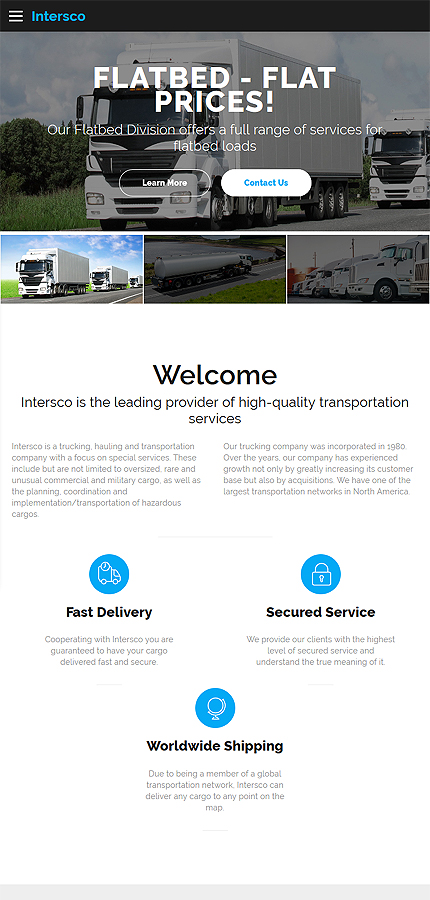**Header and Banner Description:**

On a sleek, minimalist black header positioned on the left side of the screen, three white lines form an icon indicating a dropdown menu. To the right, a vibrant neon blue logo spells out "Intersco," with the 'I' uppercase and the remaining letters in lowercase. 

**Main Banner:**

The banner below features a background image showcasing two predominantly white semi-trucks, each with a distinct black front grill. In the backdrop, lush green bushes and grass blend seamlessly with a serene light blue sky dotted with fluffy white clouds. Overlaying this scenic image is a bold white text proclaiming, "Flatbed - Flat Prices!" Beneath this in slightly smaller, non-bold white letters, a brief description reads, "Our flatbed division offers a full range of services for flatbed loads."

**Call-to-Action Buttons:**

Centered below the text are two oval buttons: 
1. A transparent button accented with a white border and featuring the text "Learn More" in white.
2. A button with a solid white background and a thin blue border announcing "Contact Us" in blue text.

**Additional Images:**

Underneath the main banner, three more images are displayed. The leftmost image is the brightest and shows another set of white semi-trucks with black grills under a blue, cloud-speckled sky, alongside grassy terrain and a patch of pavement on the left-hand side. The second image, a bit more transparent, appears to depict an industrial scene with an oil rig featuring a lengthy silver cylinder, and to the right, several semi-trucks parked in view with only their fronts visible.